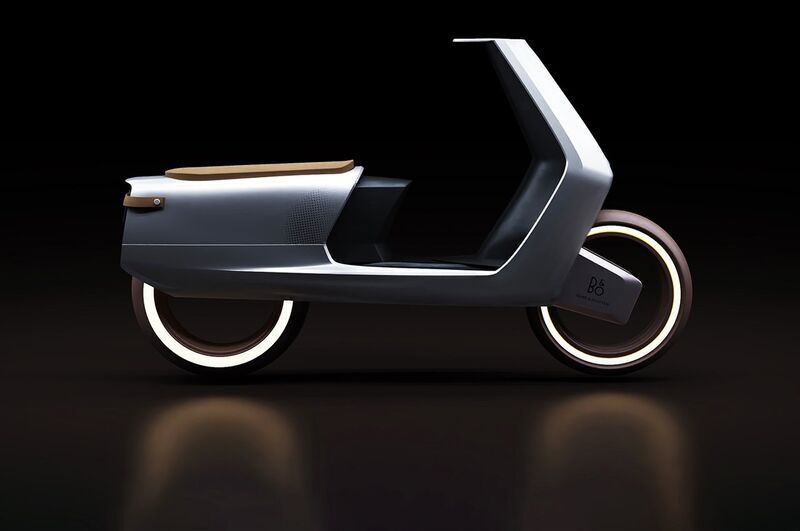The image depicts a sleek, futuristic two-wheeled vehicle, possibly an electric scooter or e-bike, set against a completely black background that creates a dark and mysterious ambiance. The vehicle boasts a metallic silver body with stylish straight lines and gentle curves that enhance its modern appearance. The black tires feature glowing inner rims, adding a high-tech touch. Notably, there are no traditional handlebars; instead, a silver stem rises from the body, suggesting an innovative steering mechanism from the middle. The vehicle is equipped with a brown seat made of plastic, offering a comfortable place to sit. A small red taillight is positioned on the back left side. The black floor beneath reflects the scooter, highlighting its glossy, mirror-like surface.